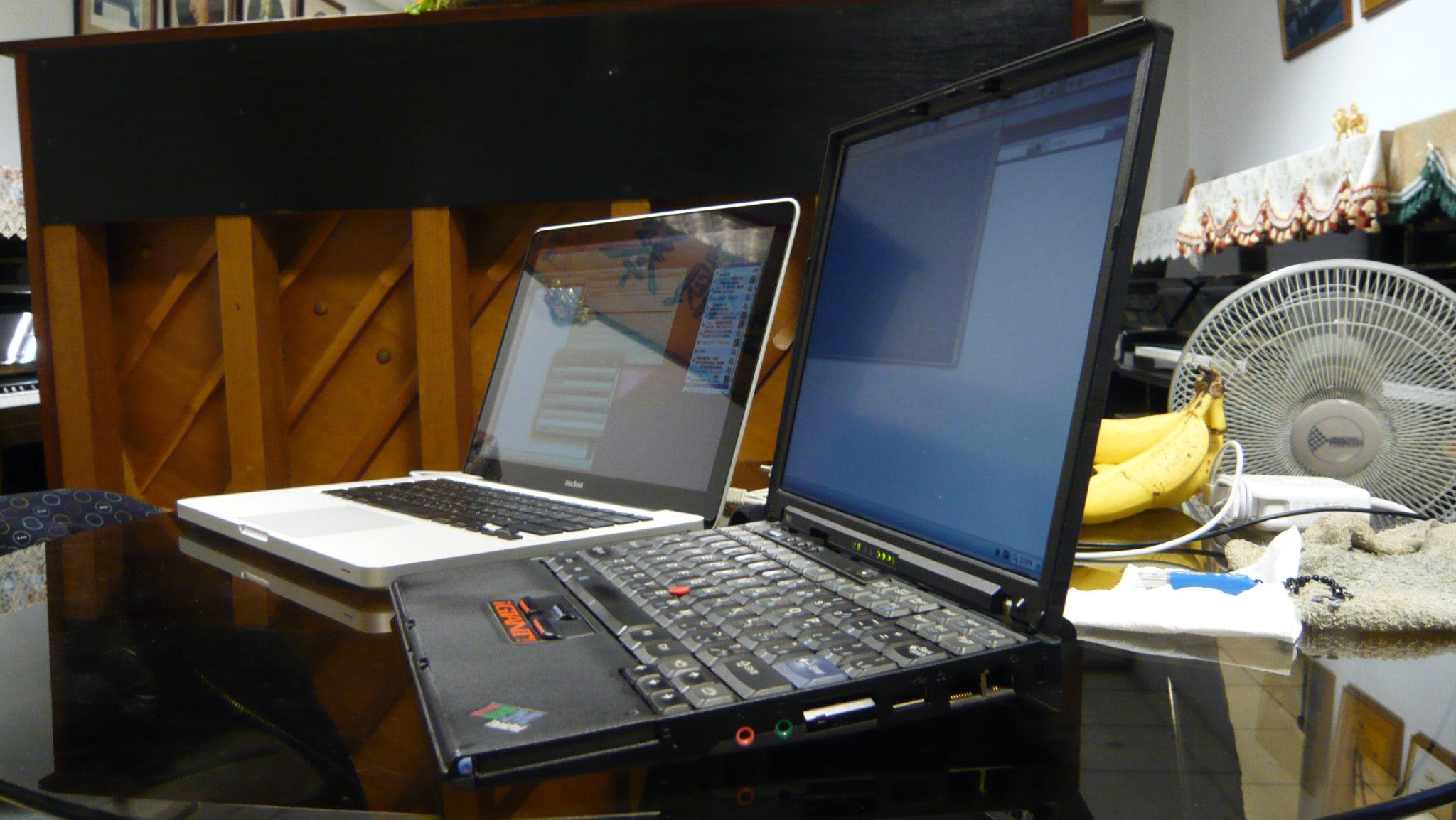In this photo, two laptops sit side by side on a round, black glass table that is shiny and reflective. The laptop on the left, which is farther from the front of the photo, is white or light gray in color and features a screen with various squares. The laptop on the right, closer to the viewer, is black with a slightly larger screen displaying a light blue background and a dark blue square. Behind the laptops, there's a white circular fan, slightly tilted, and a couple of bright yellow bananas. Also visible are a tan cloth, possibly a rag or towel, with a white folded piece of paper or a charger on it. In the background, you can see the back of an upright piano with wood paneling and some other wooden structures in front of it. A white and gray wall is also partially visible in the top right corner of the image.